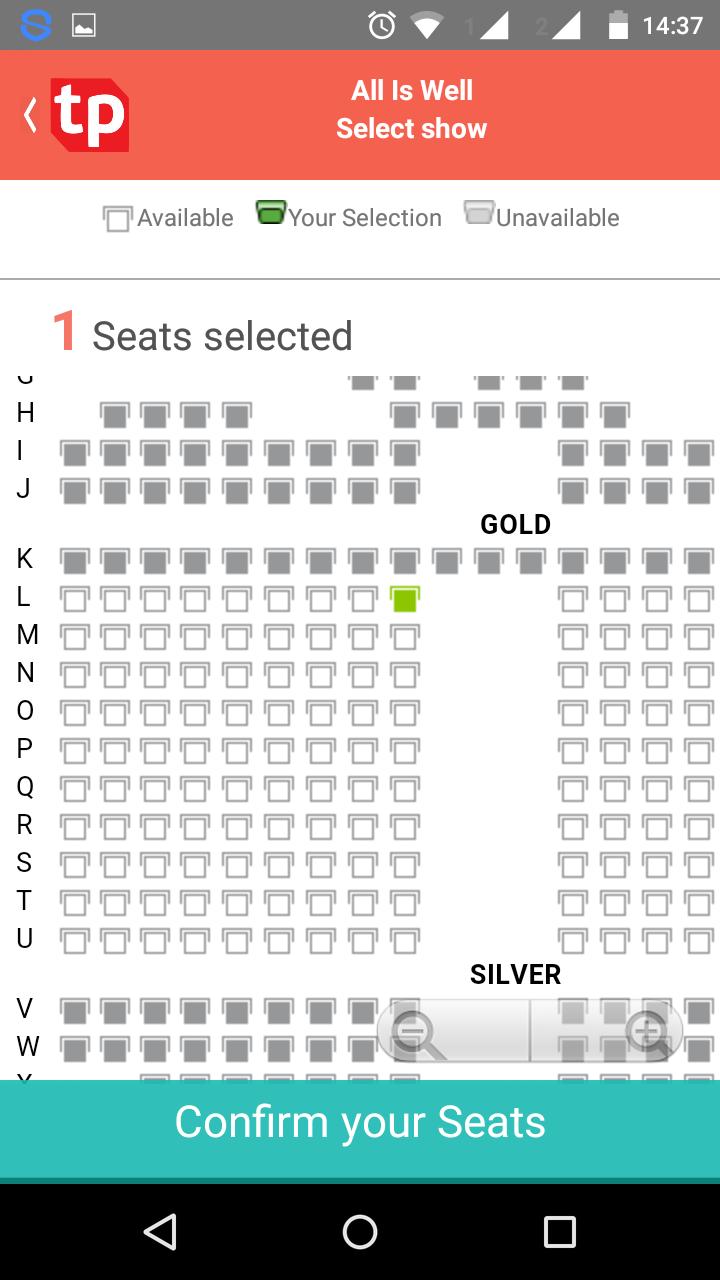The image displays a seating chart with a predominantly white background. At the very top, an alarm symbol is shown, next to a time reading of 14:37. 

The seating options are color-coded for availability: green for available seats and gray for unavailable ones. To the left, letters indicate different seating rows, though the letter "G" is partially cut off. Rows labeled "HIJ" show all seats as unavailable (gray).

Gold-colored rows labeled from "K" to "U" display a mixture of seats, with all in row "K" marked as unavailable. In row "L," there is a single seat highlighted in green, indicating it is available. 

Rows labeled "VWX" are color-coded silver. Rows "V" and "W" have all seats marked as unavailable, while row "X" shows all seats as available, although the edges are slightly cut off.

At the bottom, there is a confirmation message for the selected seats.